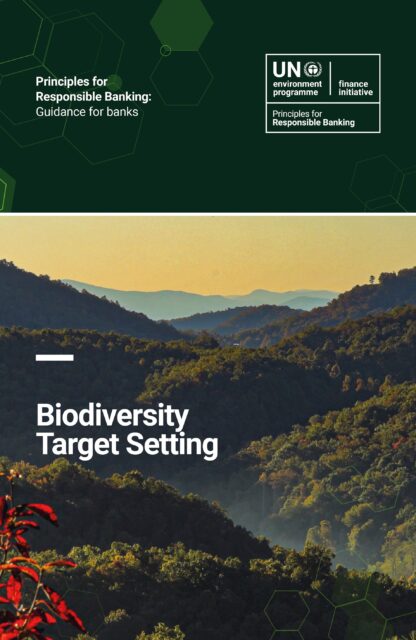The image appears to be the cover of an official UN document or report, set against a deep green background with a pattern of hexagons on the left. Prominently displayed at the top in white text, it reads “Principles for Responsible Banking, Guidance for Banks.” Accompanying these words is a square logo indicating the UN Environment Program Finance Initiative. Beneath the top section, the background transitions into a photograph of a sprawling and lush hilly landscape, densely covered in green trees and plants. Amidst this verdant scene, a red-leaved plant stands out in the bottom left foreground. The horizon showcases hills and valleys extending into the distance, set against an orange sky either from sunrise or sunset. Toward the bottom of the image, in white text, it reads “Biodiversity Target Setting.”